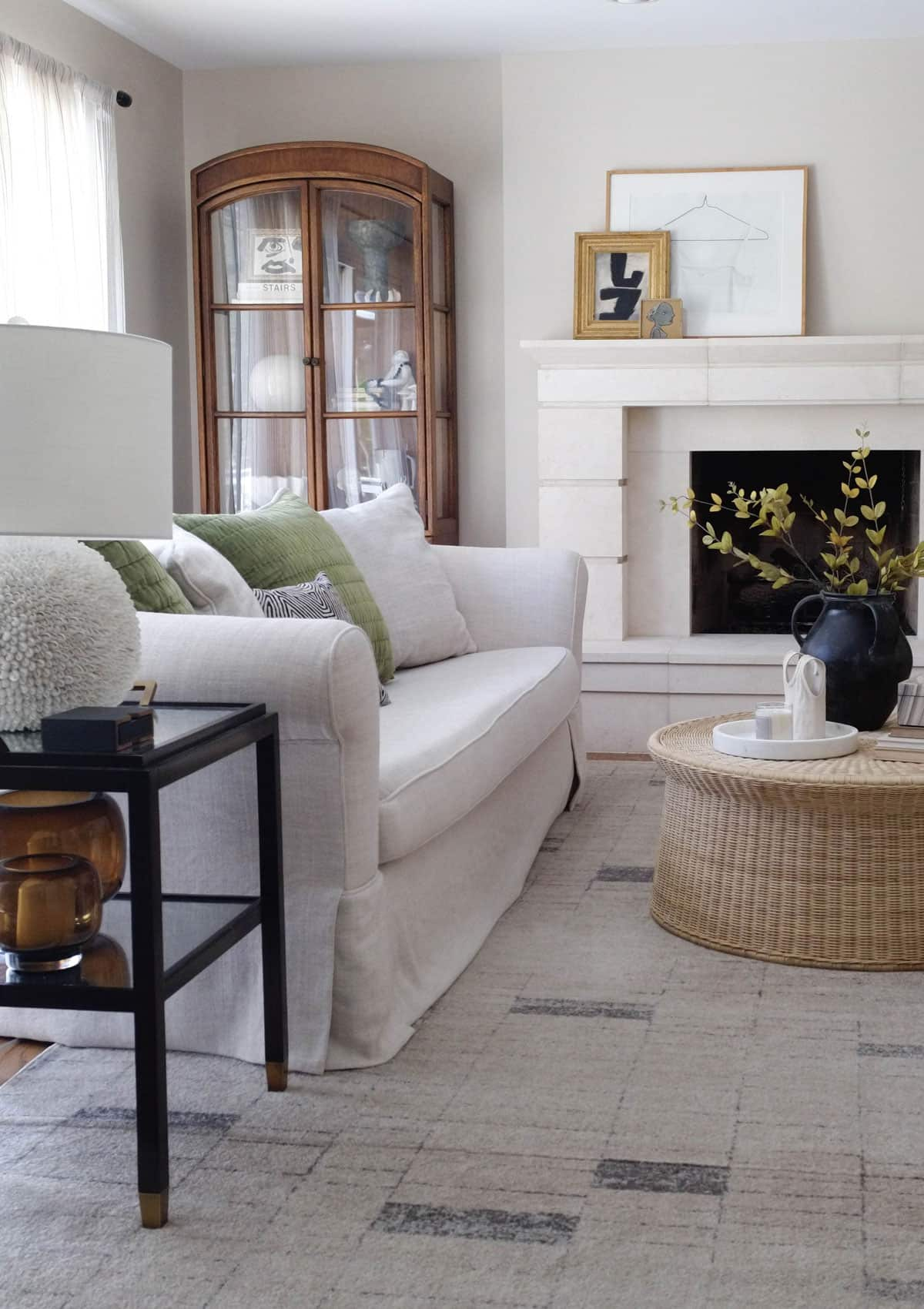This indoor photograph showcases a cozy living room, with a prominent white masonry fireplace adorned with pictures on the mantel, including a gold-framed picture and a black-and-white illustrative drawing. In front of the fireplace sits a circular wicker coffee table featuring a black metal pot with decorative green leaves, a coffee service, and a round ceramic tray with a candle. The white couch to the left is adorned with white and olive-green pillows, plus a smaller black and white pillow, complemented by a patterned rug beneath, predominantly white with small black squares. An end table with two glass shelves is situated near the couch, supporting a ceramic pitcher and vase on the lower shelf, and a remote control on the top. A wooden hutch with glass doors reveals an array of knick-knacks, including a white ball, a carved bowl, and a happy face, adding a personal touch to the room. A window with curtains stands behind the couch, letting in natural light, enhancing the serene ambiance of the space.